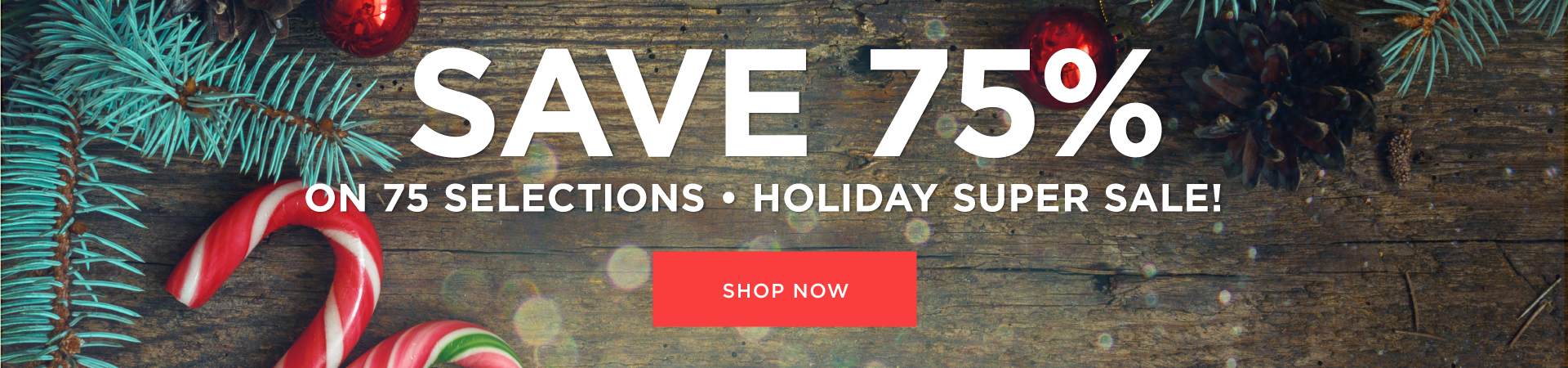The image is a screenshot featuring a brown wooden plank adorned with festive Christmas decorations, including wreaths, acorns, red ornaments, and pieces of a Christmas tree. Two candy canes can be seen, one with traditional red and white stripes, and the other with red, white, pink, and green stripes. The text on the image prominently announces "Save 75% on 75 Selections - Holiday Super Sale!" in bold white lettering. A vibrant red rectangle with "Shop Now" in white text encourages immediate action. For social media engagement, the hashtag #redsnc8 is suggested for sharing.